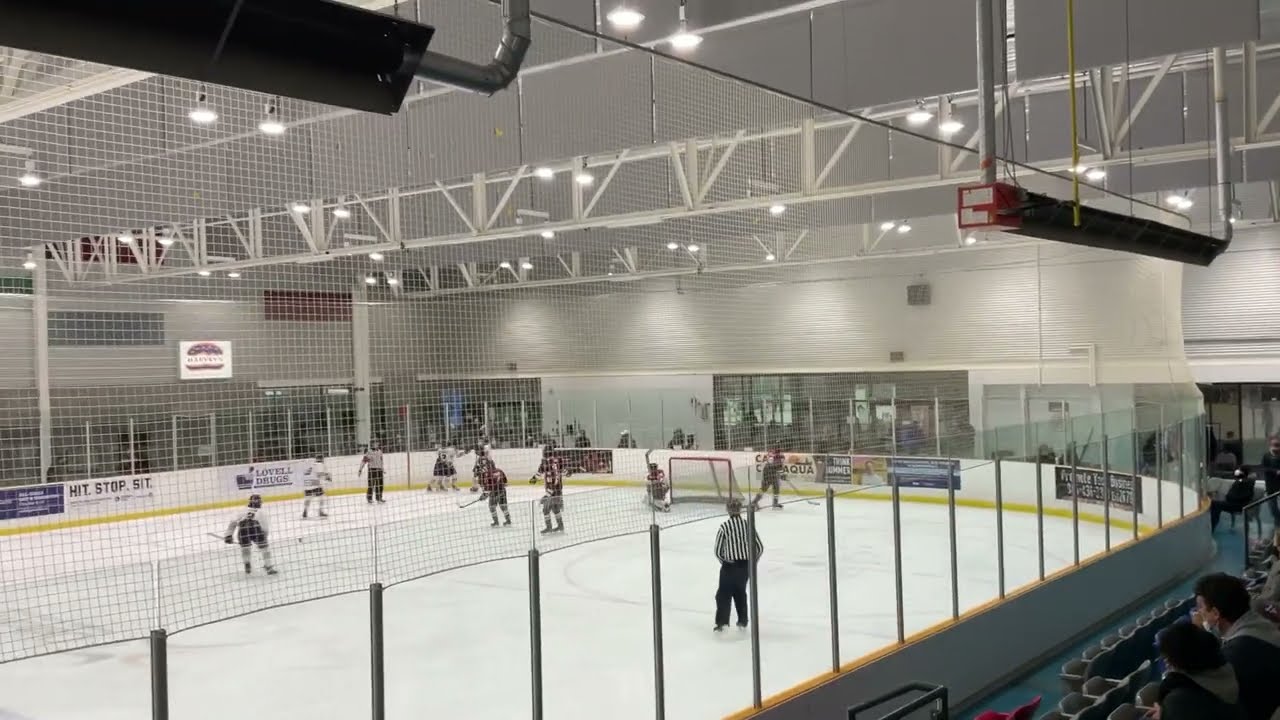This indoor photograph captures an ongoing ice hockey game viewed from the perspective of a spectator in the stands. The well-lit rink features bright white lights suspended from a high ceiling with white metal rafters. The walls of the arena are white, providing a stark contrast to the ice below. At the foreground, beginning at the lower left corner and receding into the background towards the upper right corner, we see the action on the ice rink. The rink is surrounded by a low half-wall adorned with various advertisements, including visible ones for "Lovell Drugs" and "Hit, Stop, Sit." 

Centered on the rink are players from two teams wearing red and white uniforms, actively engaged in the game with their hockey sticks bent in mid-action. A referee, distinguishable by his black trousers and black-and-white striped shirt, stands at center ice overseeing the play. Near the goal area, a goalie defends the net marked by a yellow trim encircling the rink's perimeter. 

In the lower right corner, spectators can be seen intently watching the game. Above them, black horizontal rectangular overhead structures hang from the ceiling, possibly scoreboards or additional lighting. The image vividly captures the hustle and bustle of the hockey game, the players in action, the reflective ice, and the surrounding elements that contribute to the authentic arena atmosphere.